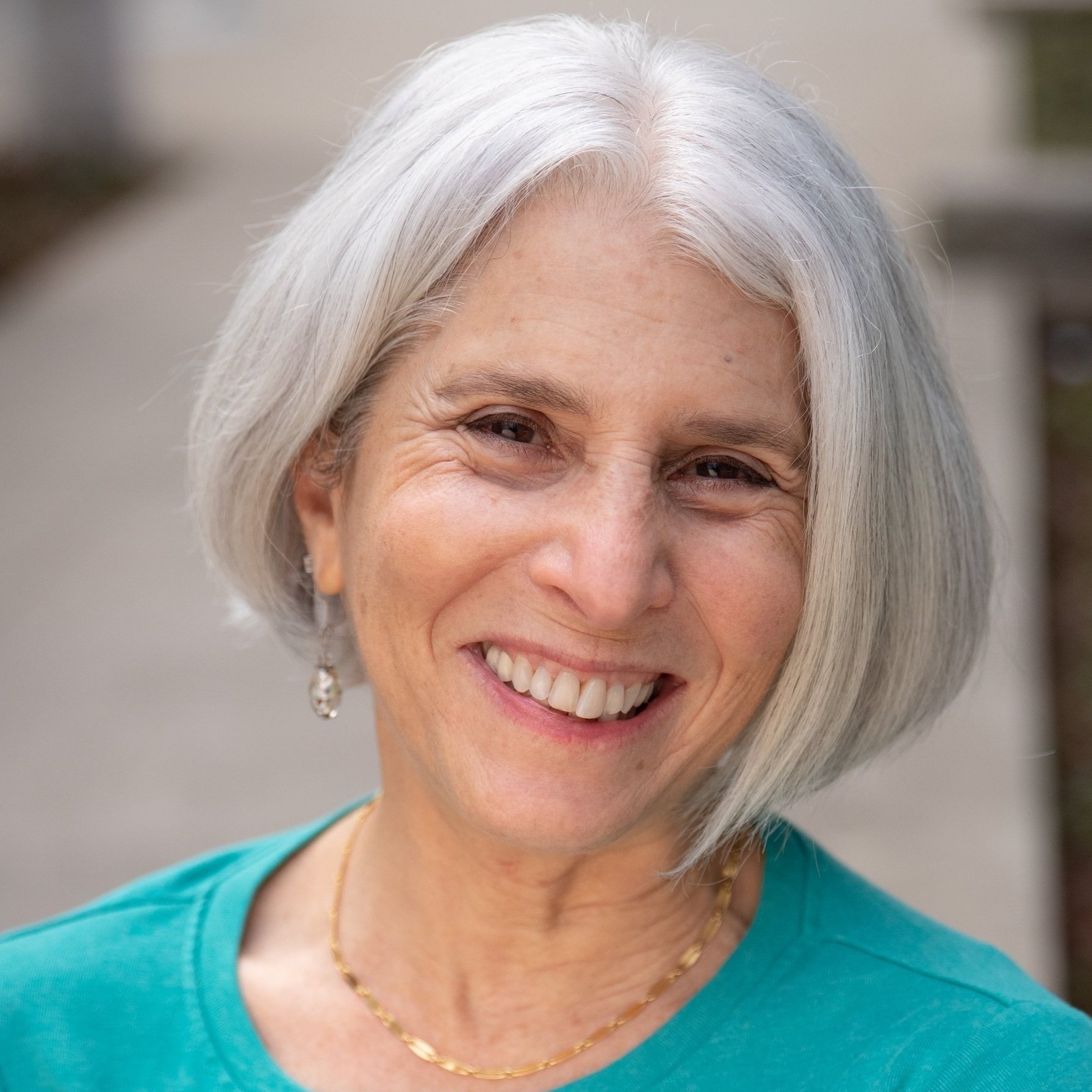This image is a detailed portrait of a Caucasian elderly woman, likely between 65 to 80 years old. She has short, chin-length, white hair styled in a soft, middle-parted bob. Her skin is fair, and she appears with very minimal makeup, save for light pink lipstick. Her smiling face reveals her upper teeth and crinkled eyes accentuated with wrinkles at the corners, showcasing her warm, brown eyes. Around her neck, she dons a delicate, gold chain necklace that sits like a choker. In her right ear, a pierced earring featuring a dangling clear, crystal pendant is visible. The background is a muted beige blur, ensuring she remains the focal point. She is dressed in a vibrant Irish green or turquoise t-shirt, contrasting nicely with her overall fair complexion.